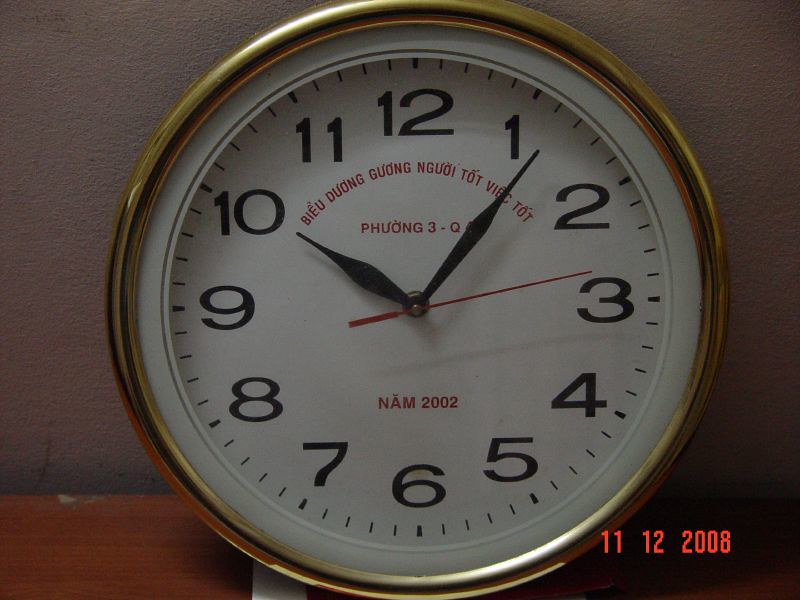The photograph features a detailed close-up of a table clock resting on a wooden surface. The clock is encased in a shiny golden rim, adding a touch of elegance. The clock face itself is white with black numerals ranging from 1 to 12, and it includes minute markers. The clock's hands are black, except for the second hand, which is red. The time displayed is 10:05, with the second hand between the 10 and 12 markers. Notably, the clock face has Vietnamese text in the upper half and "Nam 2002" written above the number 6. An additional detail includes a date, 11-12-2008, in red text located at the bottom right of the clock face. The background features a white, textured wall, contrasting with the darker wooden table the clock is placed on.